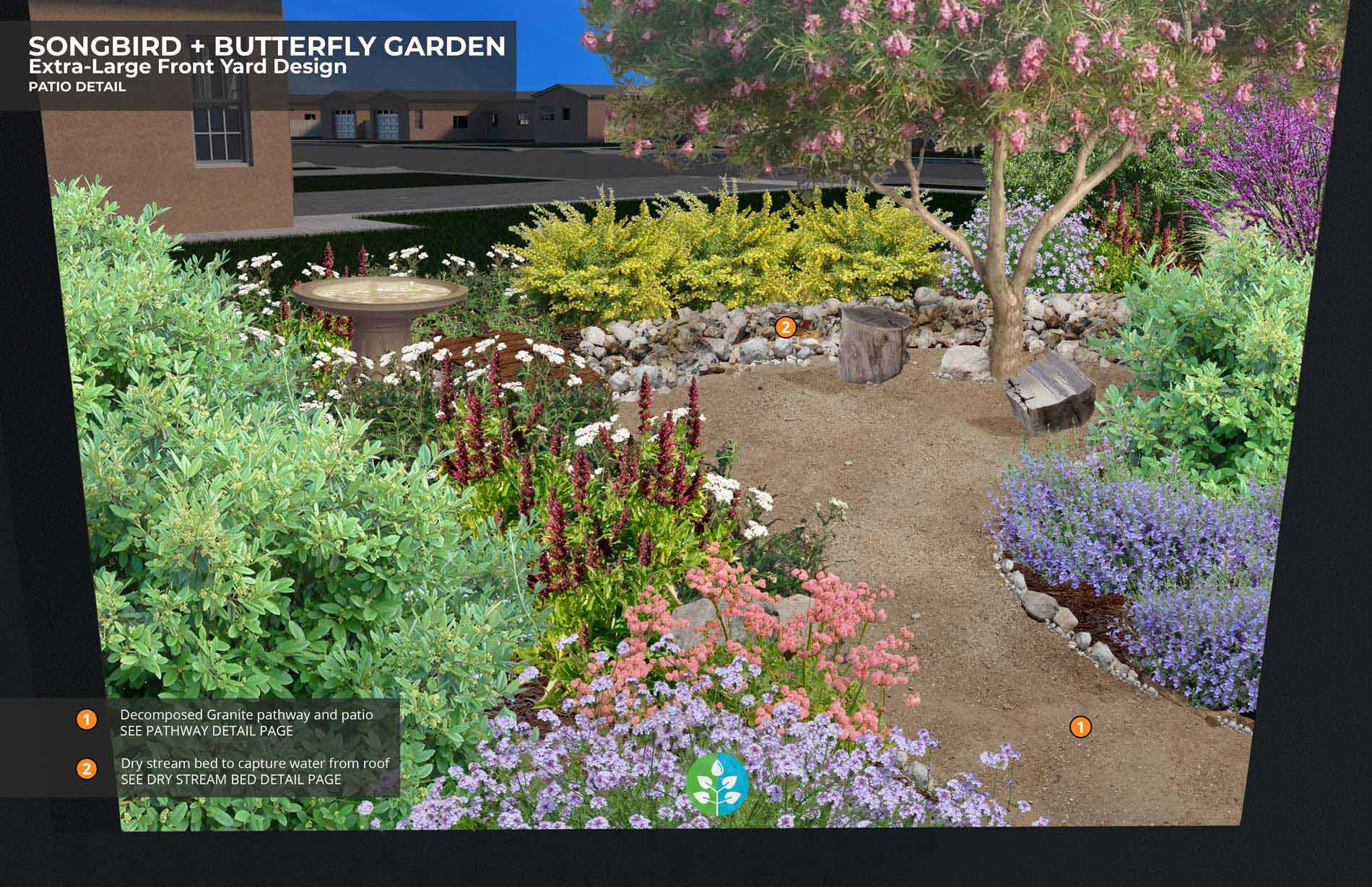This detailed digital image illustrates a conceptual design for a "Songbird plus Butterfly Garden" intended for an extra-large front yard. A transparent black rectangle in the top left corner contains white text that reads, "Songbird plus Butterfly Garden. Extra-large front yard design. Patio detail." The same type of rectangle appears at the bottom left, containing orange numbers 1 and 2 with corresponding white text descriptions: "1. Decomposed Granite Pathway and Patio. See pathway detail page," and "2. Dry Stream Bed to Capture Water from Roof. See dry stream bed detail page."

The garden features a central decomposed granite pathway that starts at the bottom right of the image and winds towards the middle. Flanking this pathway are a variety of colorful plants, including green bushes, purple flowers, pink blossoms, vertical red flowers, and blue-purple flowers. Additionally, a detailed dry stream bed designed to capture rainwater extends, adorned with rocks and subtle traces of water. A large, blossoming tree with pink flowers stands prominently in the garden, surrounded by a vivid array of green, yellow, purple, salmon, red, and pink plants. The background fades into a depiction of houses, providing context to this vibrant and ecologically focused landscape design.